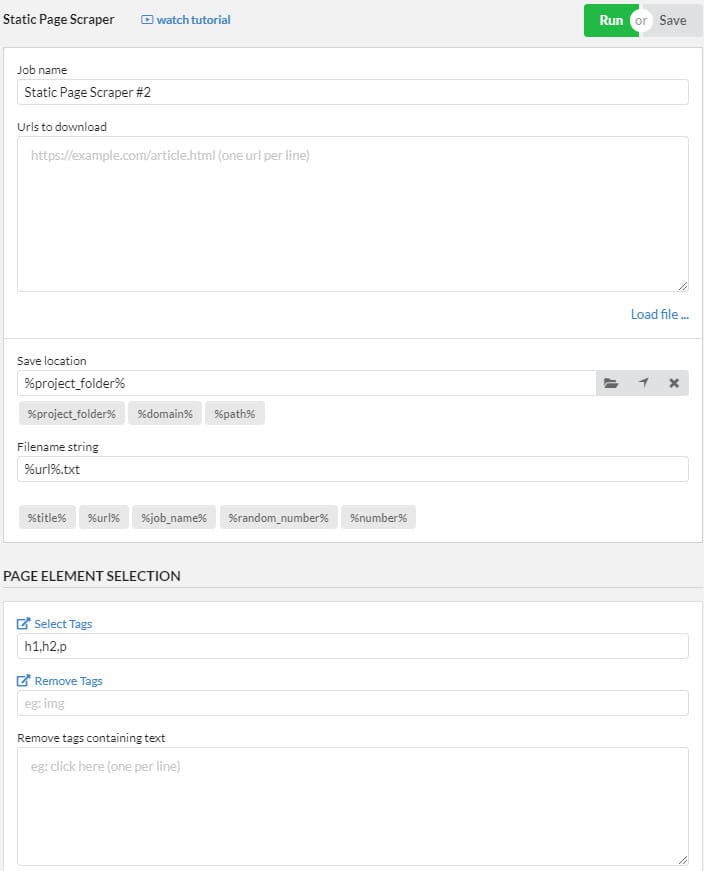The image depicts a detailed interface of a web application named "Static Page Scraper." At the top of the page, the title "Static Page Scraper" is prominently displayed. Below the title, there is a clickable blue link labeled "Watch Tutorial."

In the upper right corner, there are two green buttons labeled "Run" and "Save." Directly beneath these buttons, there is a text field labeled "Job Name" with the preset text "Static Page Scraper 2." Below this, it says "URIs to download," accompanied by a text box containing a sample website URL.

To the right and underneath this box, there is a blue link labeled "Load File." Further down, the section "Save Location" features a text field with "Project Folder" entered in it. This section includes several gray-selectable boxes below it, such as "File Name String," which currently contains some text.

Another gray section spans the width of the interface labeled "Page Element Selection," with a blue clickable option titled "Select Tags." Beside this option is a blue dropdown box with an arrow, displaying elements like "H1," "H2," and "P."

Following this, there is another section labeled "Remove Tags," featuring a dropdown box with an arrow and another box that displays the words "Remove Tags Containing Text." Instructions are given to "Click Here 1 Per Line."

The overall background of the image is white, with the only colorful elements being the blue text links and the prominent green "Run" button in the upper right corner.